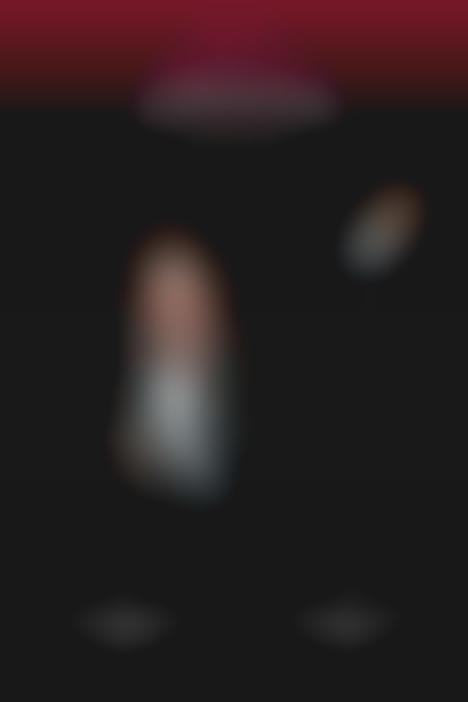In this extremely blurry rectangular image, the distinct colors and vague shapes hint at an intriguing composition. The top portion, occupying about a tenth to a fifth of the image, is a dark, blood-red blur that fades into the black background below. Within this red section, there's a hint of a triangular shape with a blend of purple and pink hues.

Just beneath this, in the middle of the image, there's a diffuse light gray or white oval shape stretching horizontally. The bottom half of the image is predominantly black, except for the middle left and right areas where faint white ovals are visible. The left side features a larger white and orangey-tan figure resembling a horn or cylindrical object, with a smaller similar shape to its upper right side. Additionally, there seems to be a silhouette-like dark shape in the middle left, possibly resembling a man with a faintly visible face in a light tan, light brown, or apricot color. A dark border frames the entire composition, enhancing the enigmatic nature of this extremely blurred scene.